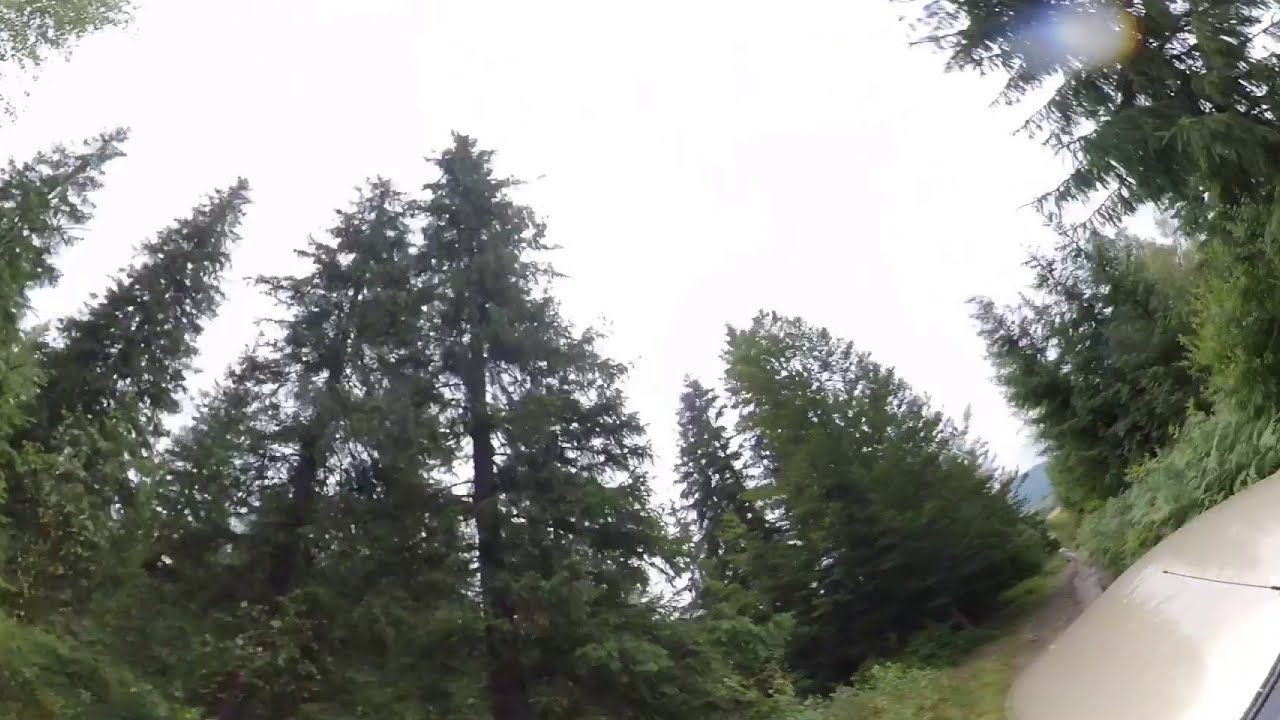From a ground-up perspective, we view a scene dominated by tall pine trees, their branches sparse and extending only a few feet from the trunk, adorned with hanging leaves. The trees on the left appear slightly taller, potentially due to the angle of the camera. The sky is a bright, blurry white, suggesting an overcast day, and obscuring any clear view of the sun. Underneath the trees, smaller bushes dot the forest floor. To the right, a dirt path slopes gently, leading through the tree-lined landscape. The lower-right corner of the image captures part of a light gray platform or possibly the top of a vehicle, indicating a viewpoint that might be from a vehicle dashboard, albeit slightly tilted. This minor detail adds a sense of immersion, as if journeying through the serene, albeit cloudy forest.